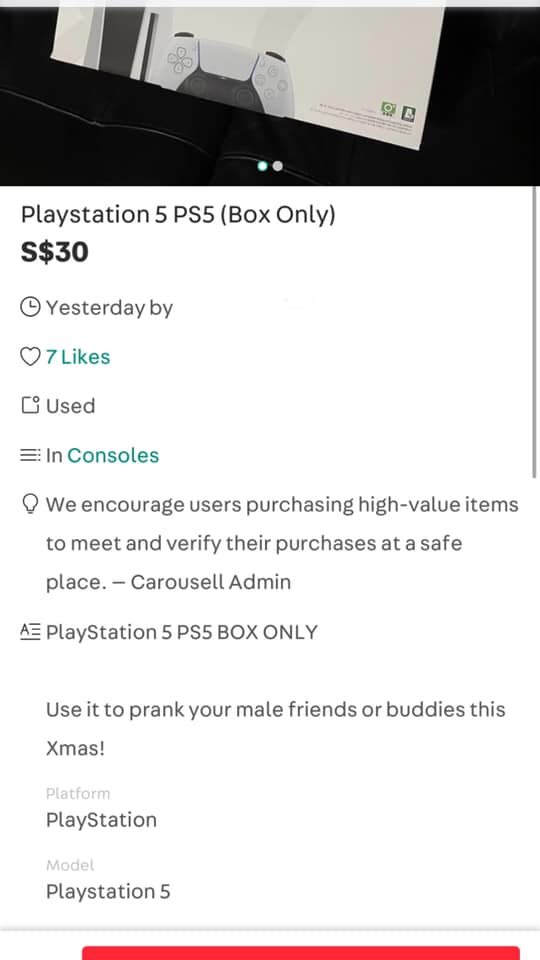The image depicts an online listing for a product described as a "PlayStation 5 Box Only" priced at $30. Interestingly, the listing has a symbol resembling an 'S' placed before the dollar sign, and it was posted the day prior. Despite seven likes indicating some interest, the seller's identity remains anonymous. The condition is marked as 'used', specifically under a console category. The platform advises users to meet in safe places to verify high-value item purchases. The description humorously suggests buyers can use the empty PS5 box to prank their friends during Christmas. The photo itself shows the cut-off bottom half of a white PS5 box, likely for the disc version, complete with an image of a controller, hinting at the era when PS5 consoles were scarce and in high demand. The listing is clearly intended as a joke, cautioning buyers that the box is empty, but it raises concerns about potential misunderstandings or disappointments for unwary purchasers.